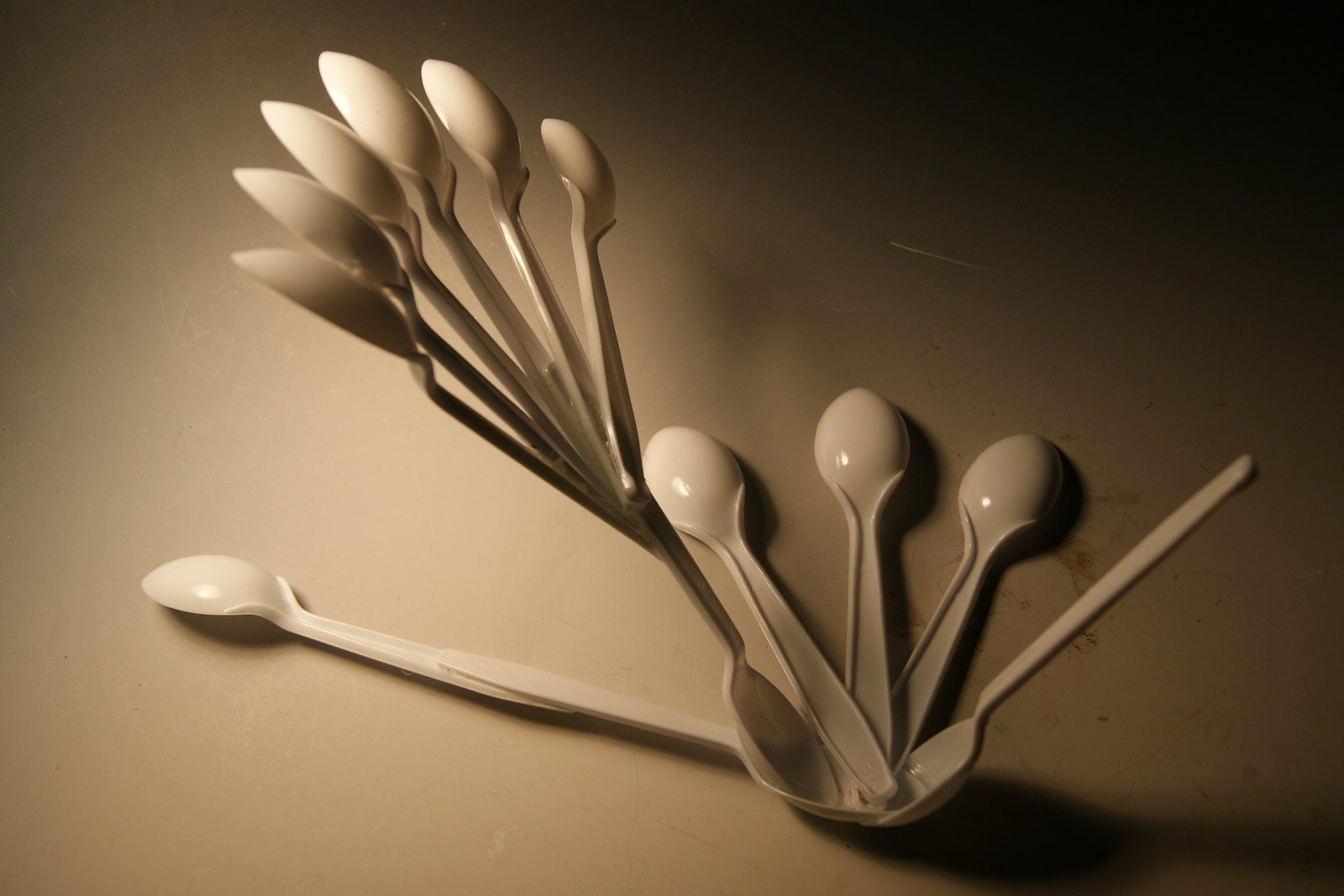The image depicts an intricate arrangement of white plastic spoons artistically displayed on a somewhat dirty, white counter that is partially in shadow, with illumination coming from the top left. The spoons are positioned in a physically improbable manner, suggesting possible digital editing or creative assembly techniques such as hot glue. Central to the arrangement is a spoon lying flat, supporting a network of six other spoons fanning out to its top, with their bowls perhaps glued together. To the right, three spoons overlap flat on the surface, with another spoon suspended above them. Additional details include scattered brown smudges or stains on the counter, particularly under some of the spoons, and the overall low-resolution quality of the image, which lends a darker appearance to the top right and lighter to the lower left areas.